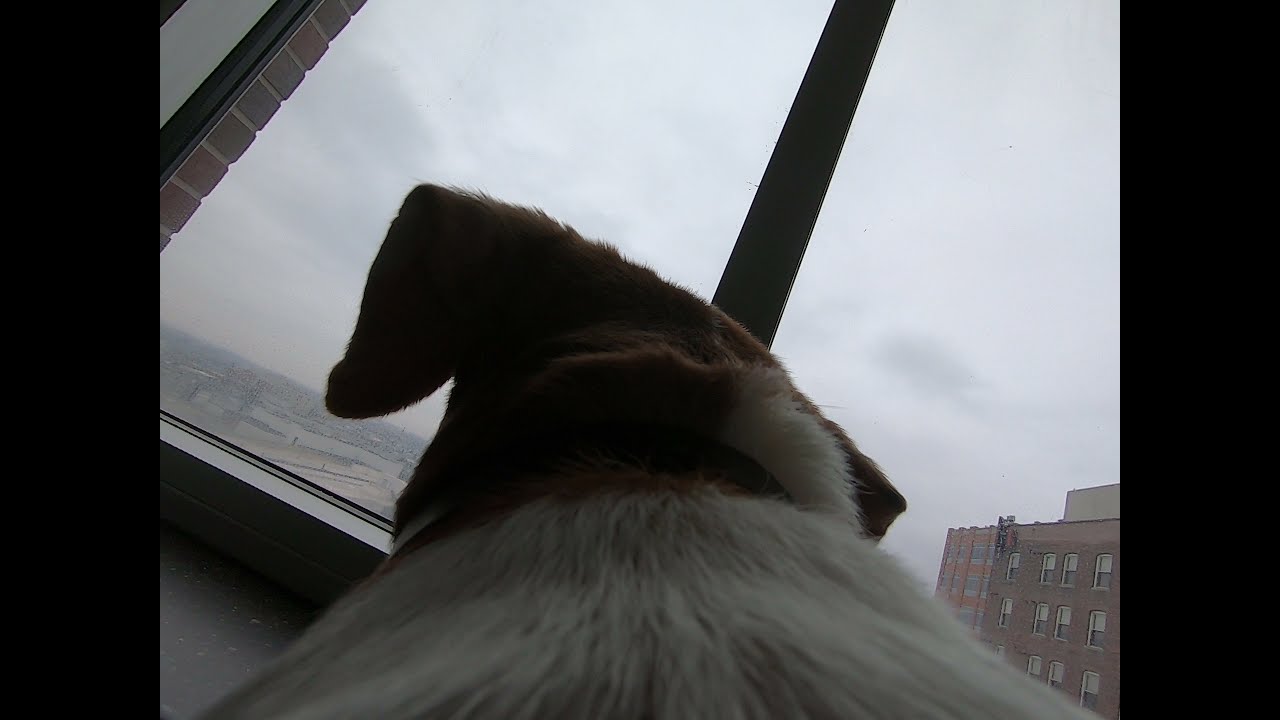In the image, a dog with a white and reddish-brown coat, identifiable by its collar, is seen from behind as it looks out a large glass window. The dog occupies the bottom center of the frame. The backdrop reveals a grey, overcast sky, suggesting a stormy look as the clouds loom heavy. To the bottom right, above the dog, part of a brick building with brown and orange bricks is visible. Further to the right, another brick structure is discernible, perhaps part of the same building. The scenery outside the window, though slightly blurry and possibly wet from rain, hints at a congested neighborhood, possibly in a city with a hint of greenery and soft hills in the distance. The overall scene presents a serene yet somewhat dreary atmosphere, captured from an indoor vantage point on what seems to be a rainy day.